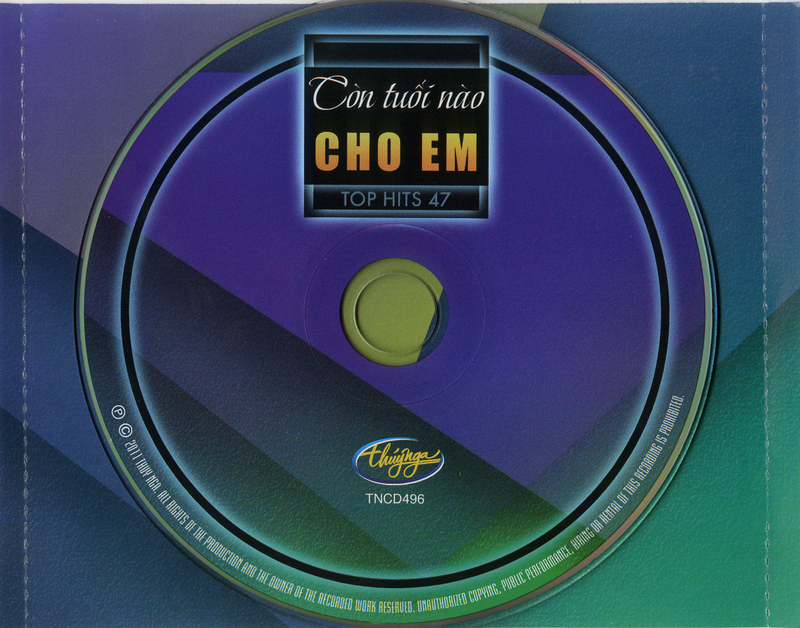The image is a colorful cover for a music record or CD titled "Contwee Now." The design prominently features a circular outline resembling a record with multiple concentric circles. At the center top, a black square contains text, some of which are in white and orange, and "Top Hits 47" is printed below. The title "Choem" appears in yellow text, beneath which the name "Thunya" is also in yellow, followed by "T-N-C-D-4-9-6" in white. The background of the cover is adorned with a vibrant mix of purples, blues, and greens with abstract geometric figures. At the bottom, along the circular edge, is a detailed copyright notice from 2011, warning against unauthorized copying, public performance, hiring, or rental of the recording.